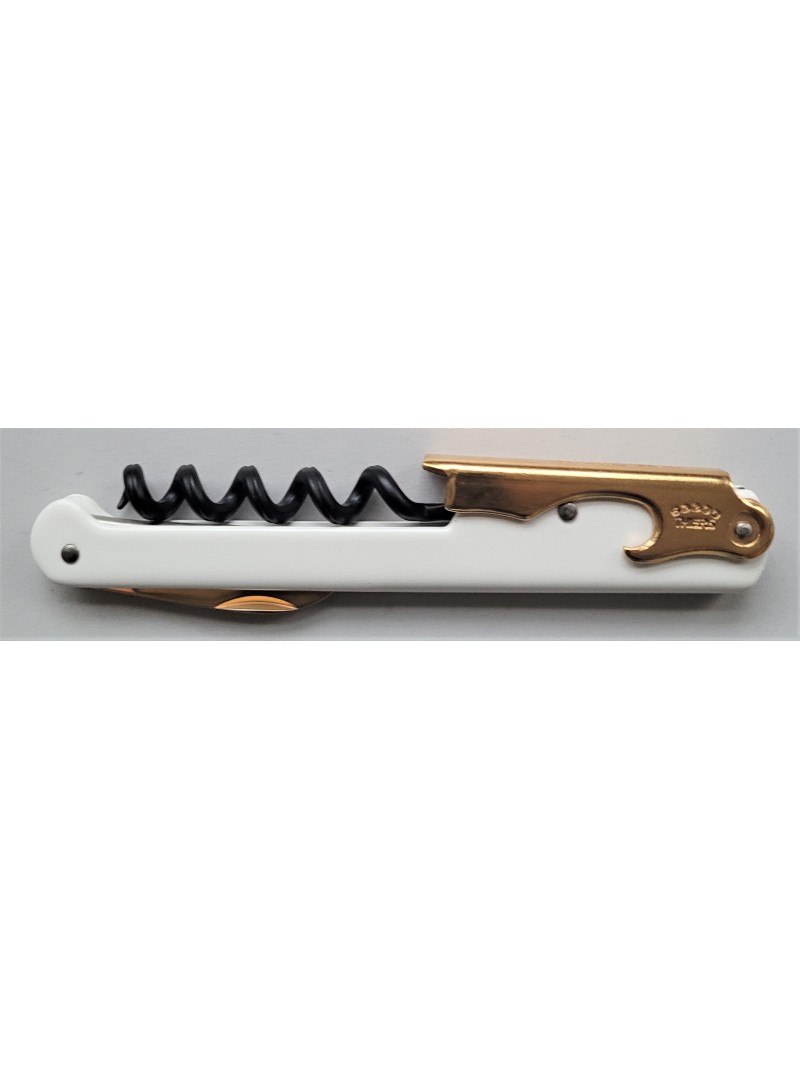The image depicts a folding multi-purpose wine opener, commonly known as a Swiss knife. The tool has a sleek, white body, complemented by a luxurious copper-colored handle. Key components include a black corkscrew, a short blade that is copper-colored on the inside and brown on the outside, and a brass-colored bottle opener folded against the upper right-hand side. The knife blade is situated on the lower part of the tool and is about two-thirds the length of the corkscrew. The entire tool is mounted against a light gray background with a thin shadow along the bottom edge, suggesting overhead lighting. Additionally, the name, which appears to be "Gadsby" or "Gabby," is stamped on the copper section, along with dark gray studs, contributing to the tool's sophisticated appearance.